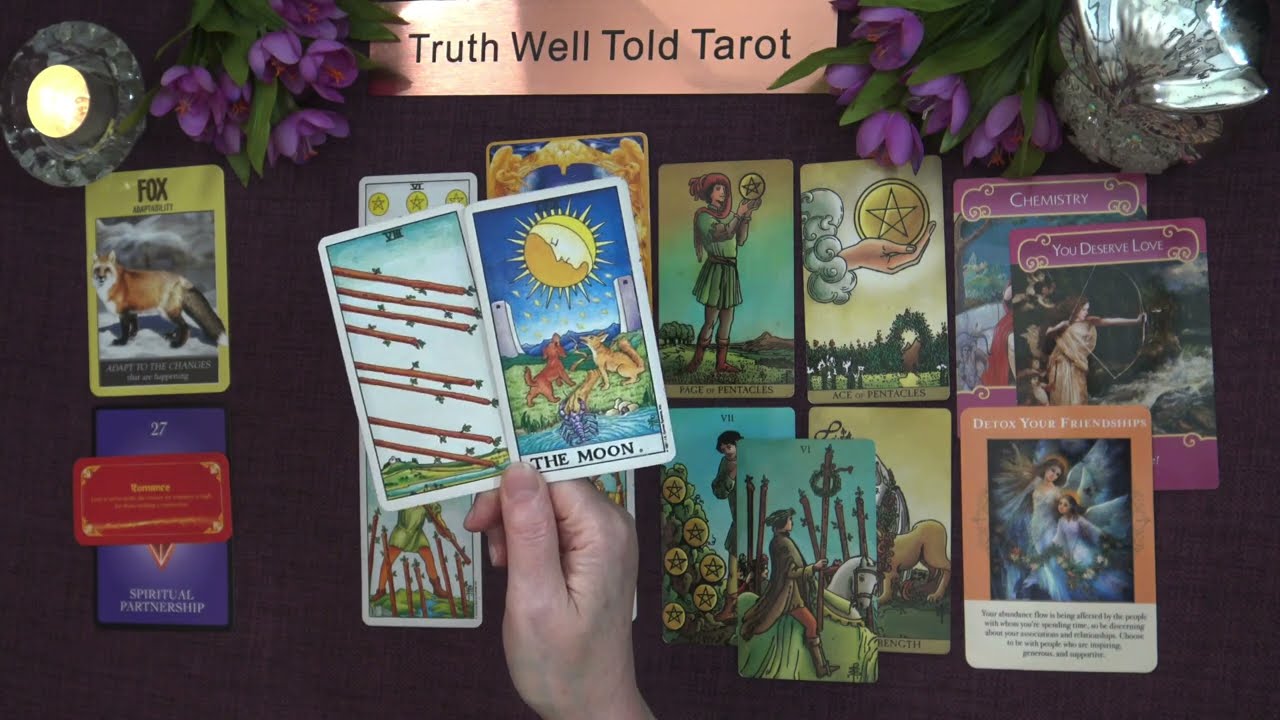In the image, a hand slightly left of center holds up a tarot card titled "The Moon," featuring a striking depiction of a moon with a face, likely a woman, looking down as dogs or foxes howl up at it. Surrounding this focal point, several tarot cards are laid out, each teeming with rich, fantasy-inspired illustrations. To the left, another card shows an image of sticks, while a separate card features a vivid depiction of a fox. Behind the hand-held card, a series of other tarot cards displays various scenes, including characters like a medieval figure in green holding a glowing sphere with a star, and an image of someone riding a horse. To the right, three specific cards stand out, each with purple accents and text: the bottom one reads "Detox Your Friendships" alongside an image of angels, the middle one says "You Deserve Love," featuring a woman with a bow and arrow accompanied by another figure, and the top card is labeled "Chemistry." The scene is crowned by a sign at the top reading "Truth Well Told Tarot," flanked by purple flowers. Additional decor includes a lit candle in the top left corner and an owl statue in the top right corner, completing this intricate and captivating tableau.